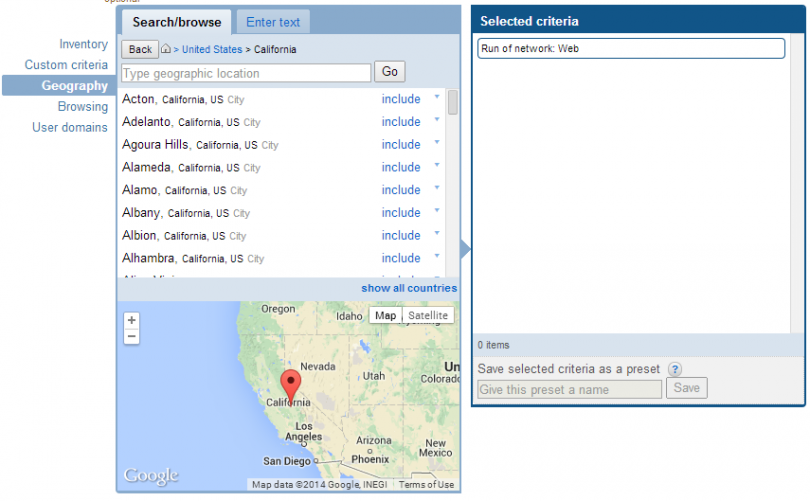The image showcases two screenshot windows of a geographical search interface. In the first window, a search bar prompts users to "Search, browse, enter text" with a filter set to "United States, California" and instructs the user to "Type geographic location." Below this prompt, a map of the United States is displayed, highlighting various Californian locations starting with the letter "A," including Acton, Calgary Hills, Alameda, Alamo, and Albany. On the left side of this window, several menu options are written in blue, such as "Inventory," "Custom Criteria," "Geography," "Browsing," and "User Domain," with a blue highlighter bar indicating selection.

The map itself features state borders and labels for neighboring states, which include Oregon, Idaho, Nevada, California, Arizona, Utah, Colorado, and New Mexico, as well as the Pacific Ocean to the west. The map appears to be from Google Maps, identifiable by its distinct style.

The second window on the right seems to be a selection box where the chosen geographic locations and criteria are saved. It appears to have a functionality such as “Run network web,” enabling further actions based on the selected geographic data.